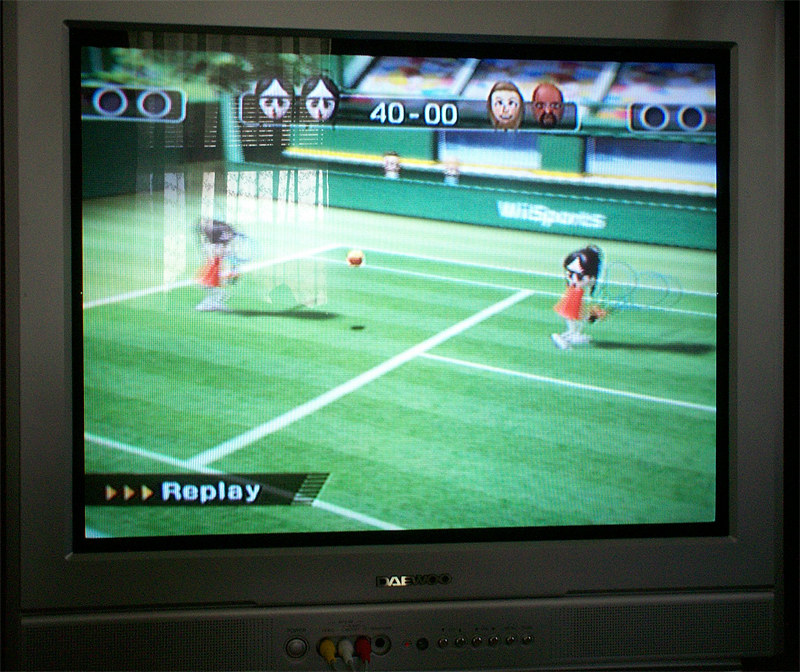The image depicts a screenshot from a Wii Sports tennis game displayed on an old Daewoo television, set in a living room. The TV, characterized by its gray boxy frame and front control buttons, shows a classic green tennis court with white stripes. The score at the top reads 40-0, and the screen displays a moment from the game with "Replay" indicated in white letters at the bottom left. Centered on the screen are two female characters, both with their hair in buns and wearing glasses, dressed in matching reddish-orange skirts and white shoes. They are positioned on the left half of the court, both poised with tennis rackets as a ball is mid-air between them. In the background, the text "Wii Games" is visible, along with a spectator stand that includes four distinct characters: likely twin spectators on the far left, followed by a black gentleman with a mustache, and a white woman with brown hair.